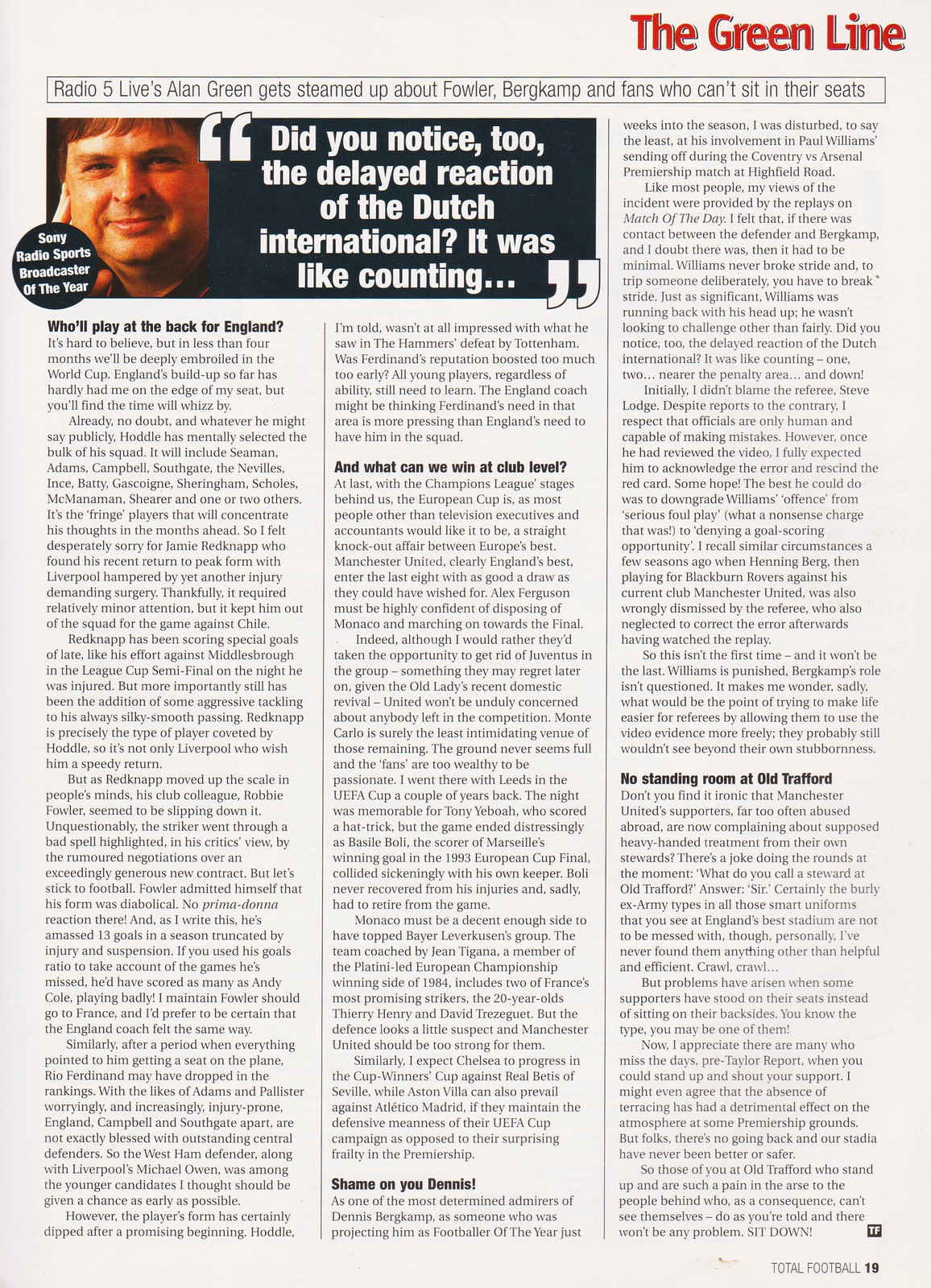The image depicts a portrait-oriented magazine page, featuring a section dedicated to soccer or football club content. Dominating the top right of the page, in bold red text, is the headline "The Green Line," set against the typical off-white or light blue-gray background common in magazine publications. To the left of this headline, spanning the top two columns, is a photograph of a man gazing and smiling at the viewer. Accompanying the image, a large white quote reads: "Did you notice, too, the delayed reaction of the Dutch international? It was like counting..." Below the man's photo, a black circle contains white text declaring, "Sony Radio Sports Broadcaster of the Year."

The layout consists of three columns of black text, each featuring bolded headlines followed by related articles. Noteworthy headlines include "Pool Play at the Back for England?" at the top of the first column, "And What Can We Win at Club Level?" in the middle column, and "No Standing Room at Old Trafford," located a bit past halfway down the third column. At the bottom of the middle column, another headline states, "Shame on You, Dennis!" while the bottom right corner of the page notes, "Total Football, page 19." The page's top text, "Radio 5 Live's Green gets steamed up about followers, Kana Bergkamp, and fans who can't sit in their seats," sets the stage for the articles and the man's quoted sentiments.